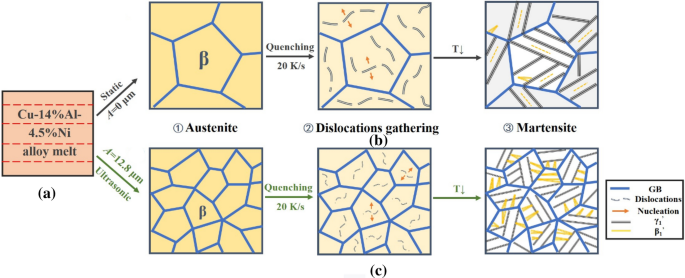The image depicts a detailed scientific graphic illustrating a chemical reaction and phase transformation in a metallurgical process. It is organized into six squares that each represent different stages of the transformation. The process begins with an alloy melt containing 14% copper and 4.5% nickel, indicated in the top left. From this initial state, the graphic shows the alloy undergoing static treatment, denoted by "A=0," and progressing through ultrasonic stimulation.

The sequence follows the transformation from austenite, through a quenching process at a rate of 20 kilos per second, leading to dislocation gathering. This transformation is classified into two main phases: first and second stage dislocations. The end stages feature the formation of martensite, depicted in blue with intricate lines representing structural changes.

The graphic includes various colors and lines to signify different elements and transformations. Yellow and beige indicate early stages, transitioning to blue and cream, then finally to blue, black, white, and yellow to represent martensite. A key on the right side decodes these symbols: dark blue lines indicate grain boundaries (GB), dashed lines represent dislocations, arrows show nucleation points, and black or gray lines represent gamma phases, while yellow lines denote beta phases.